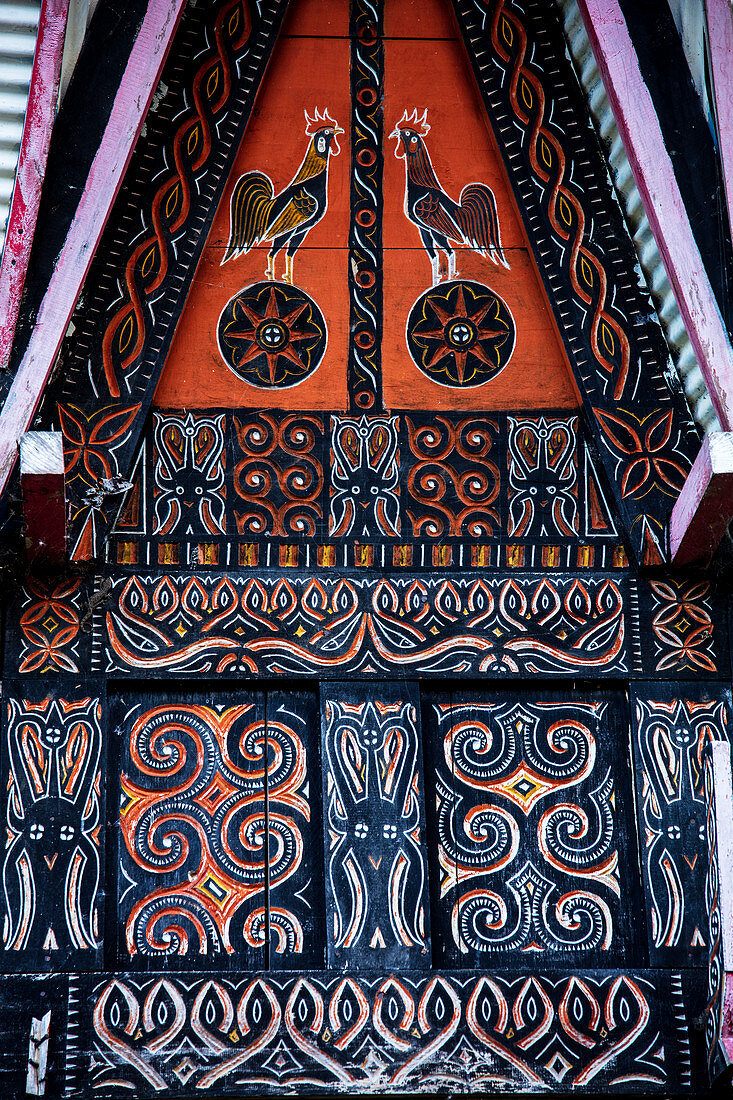This detailed and ornate outdoor structure, possibly a temple or a mural adorning a building's side, captures the eye with its intricate and vivid design. The top of the structure features an A-frame roof with distinct pink wooden pieces, beneath which lies an orange triangle divided into two panels. Each panel showcases a rooster, with the left one painted yellow and the right one in red. Both roosters stand atop circles adorned with orange flowers that have a white interior and a cross in the center.

Below these roosters, the structure displays five panels with complex designs. Three of these panels feature creatures resembling squid with ears and arms, while the remaining two showcase snail-like figures. Further down, there is a panel that gives the appearance of candles. This is followed by another set of five panels mirroring the squid and snail motifs described earlier. At the very bottom, a final panel again depicts what looks like candles.

Overall, the primary colors in this artistic masterpiece are orange, black, and white, with accents of red and blue highlighting the details in the floral and spiral patterns. The combination of roosters, floral motifs, and imaginative creatures creates a visually captivating and richly detailed work of art.